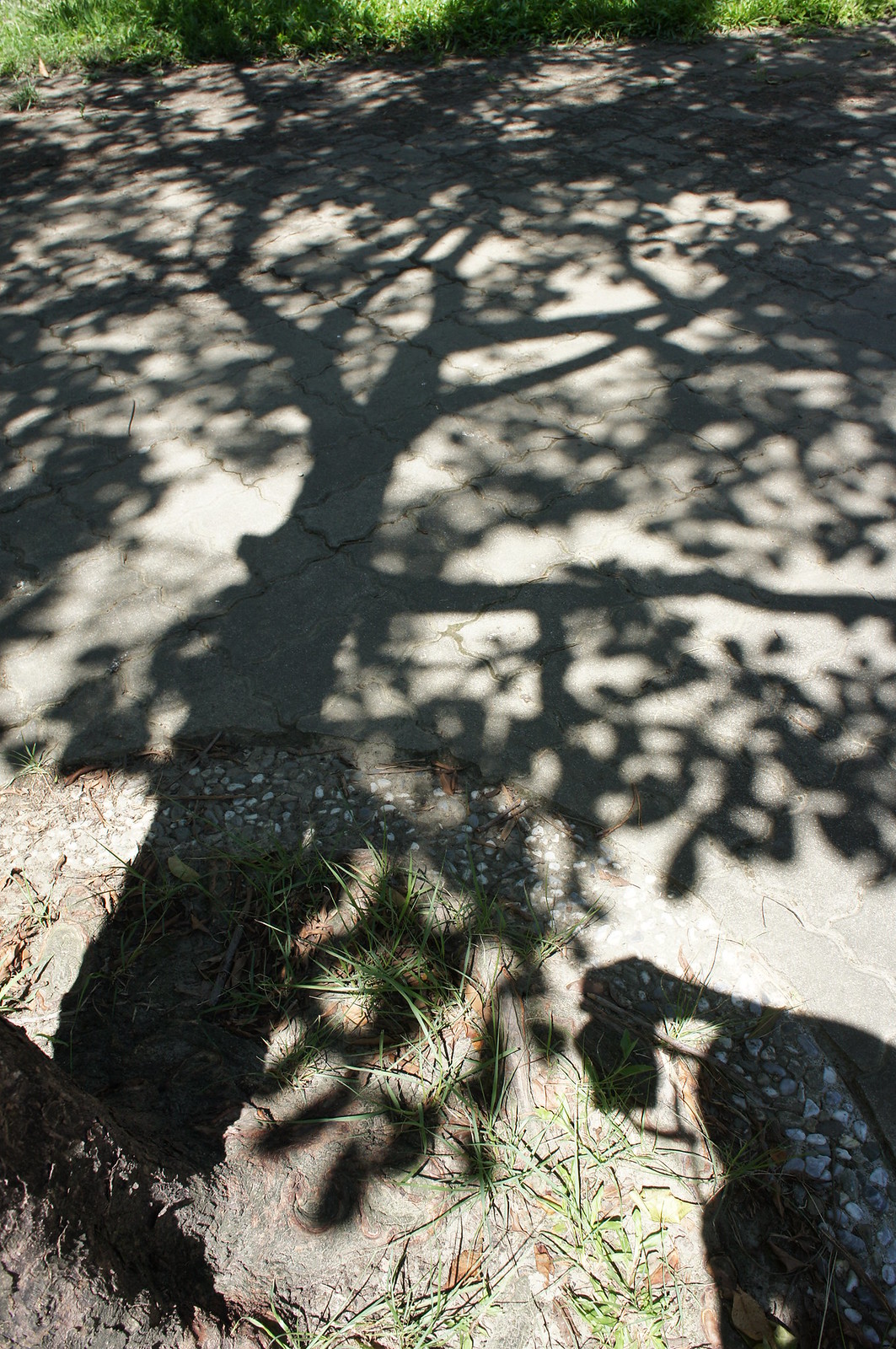This is an outdoor top-down photograph taken in the middle of the day, predominantly featuring a cracked and broken asphalt road. In the bottom left corner, a hilly area with gravel and sparse grass can be seen, along with the trunk of a tree. The tree casts a noticeable shadow across the ground, revealing detailed branches and leaves. Near the top of the image, a thin line of overgrown, bright green grass is visible. In the bottom right corner, the shadow of the photographer is present, showing them wearing a camera around their neck and holding it above their head. The colors in the image include shades of green, gray, white, black, brown, and orange. No text is visible in the photo.